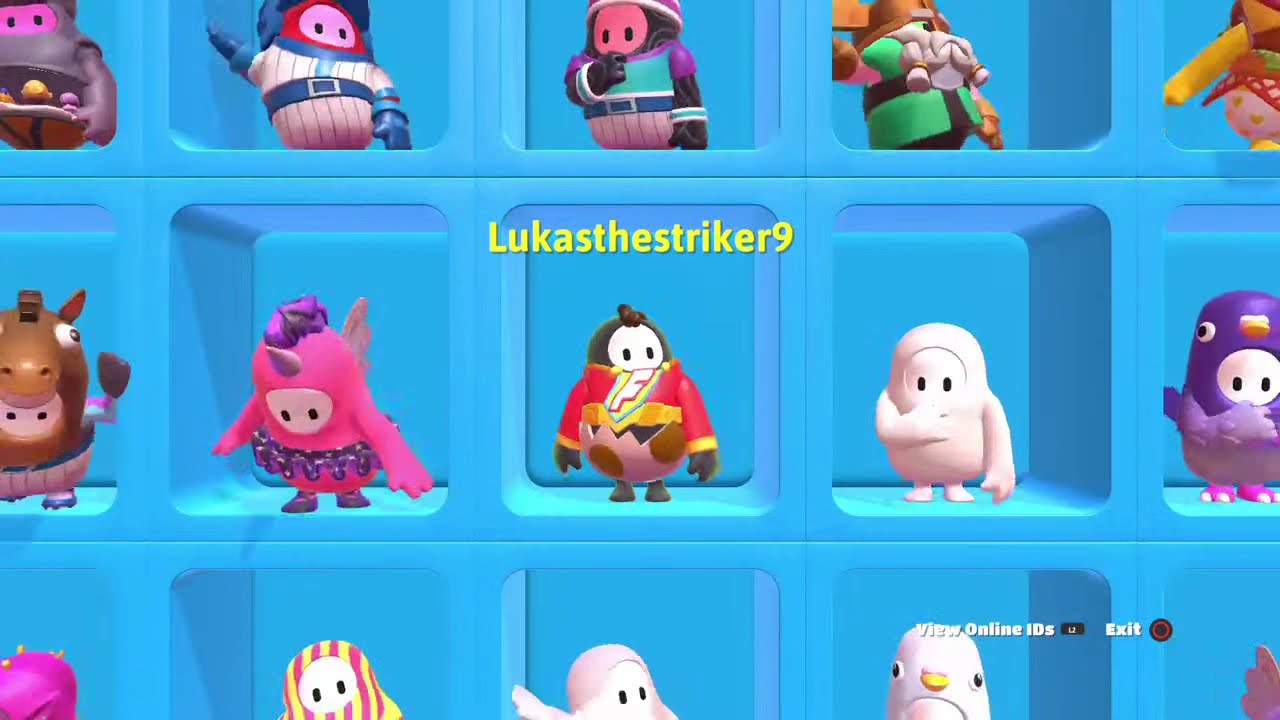This digital artwork portrays a vibrant, blue wall divided into square-shaped compartments, each housing a colorful character. There are approximately 15 figures, resembling animated children's toys or video game characters, dressed in various uniforms and outfits. Each character has two hands, two legs, and two eyes, and they all strike different poses, adding dynamic energy to the scene.

In the center of the image, the words "Lucas the Striker 9" are prominently displayed in yellow. Towards the bottom right corner, white text reads "view online IDs exit." Notable figures include a character in a wetsuit, another in striped clothing, a green-bearded figure, a penguin, a unicorn-like creature, a horse, and various bird-like characters. The compartments are arranged in three rows, with the bottom row partially cut off, showing only the heads and parts of the figures.

This detailed layout and the diverse, vividly colored characters suggest the image might be related to a video game, bringing a playful and engaging visual experience.